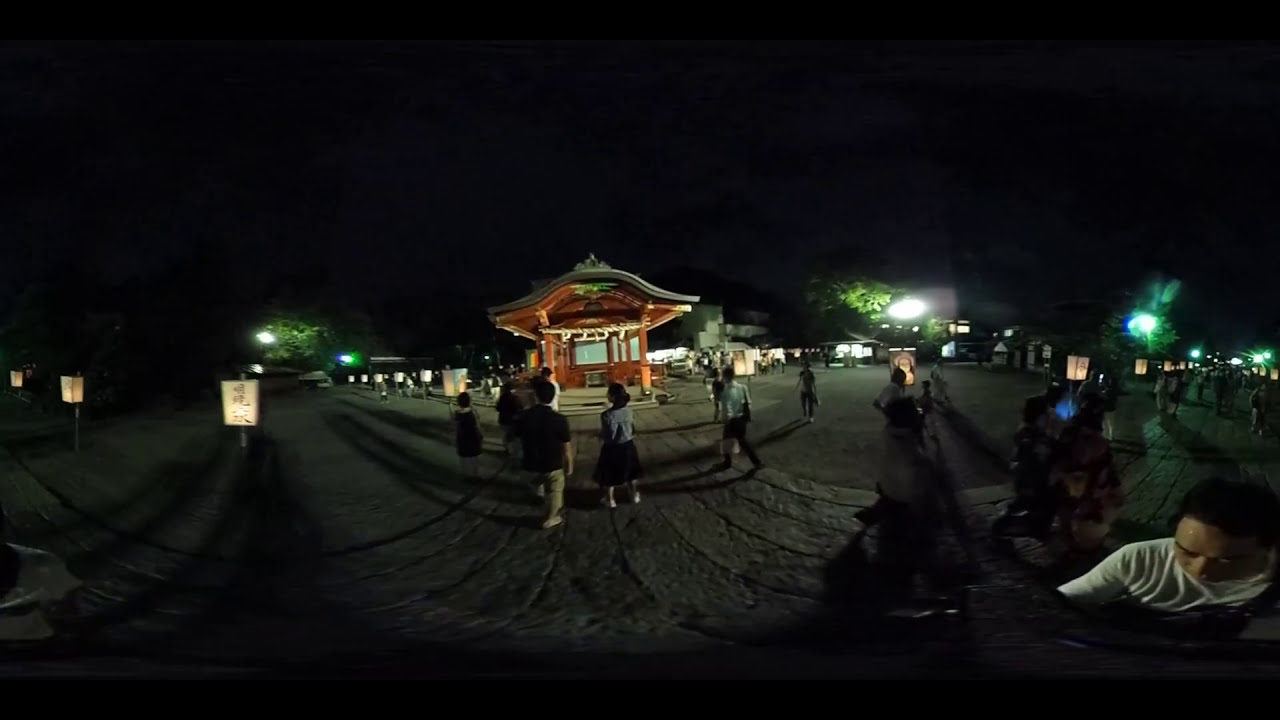The image captures a panoramic nighttime scene featuring a small, Asian-style shrine or pavilion situated in the center of a public square. The shrine, constructed of medium-colored reddish-brown wood with a black curved roof, stands prominently against a solid black sky. It features two columns at its front and a few steps leading up to it, with several green trees visible in the background, some illuminated by streetlights while most remain shrouded in darkness. The square itself has a textured stone or paved walkway, and is adorned with evenly spaced lanterns bearing Asian writing. 

A crowd of six or seven people, dressed mostly in dark attire, have gathered around the pavilion, their backs turned towards the camera. One notable individual, wearing a white shirt and having short black hair, stands in the lower right-hand corner of the image, facing the camera. This person and the people around give an impression of a summer night due to their light, casual clothing. The scene is bathed in a gentle illumination from nearby streetlights and lanterns, creating a serene and culturally rich atmosphere.